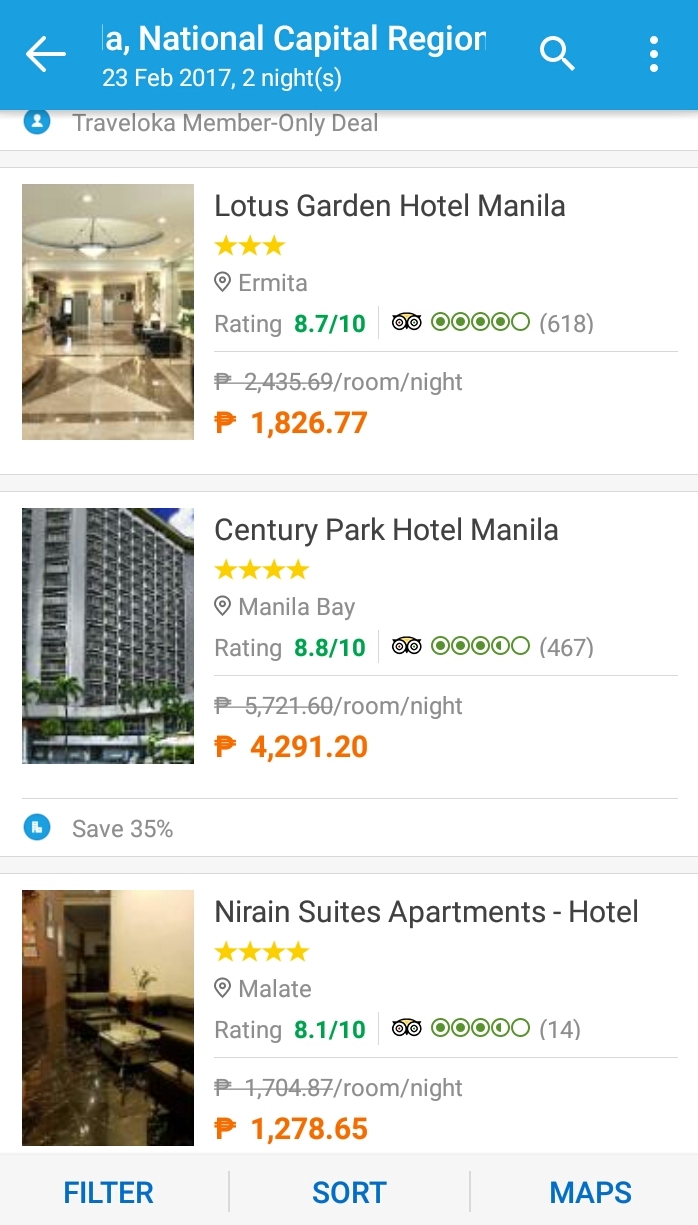A screen capture displaying the details of three different hotels is shown. At the top of the screen, a blue bar features the text "National Capital Region. 23 February 2017. Two nights" written in white. Below this bar, the first hotel is showcased: an image of a large lobby with a luxurious chandelier, shiny polished floors adorned with a large, geometric design in black and beige. To the right, the text reads "Lotus Hotel, Lotus Garden Hotel Manila." Below it, an image of a tall high-rise hotel appears with the adjacent text "Century Park Hotel Manila." The final image, at the bottom, presents the interior of a hotel suite with pristine white walls. To the right of this image, the text "Niran Suites Apartments Hotel" is displayed.